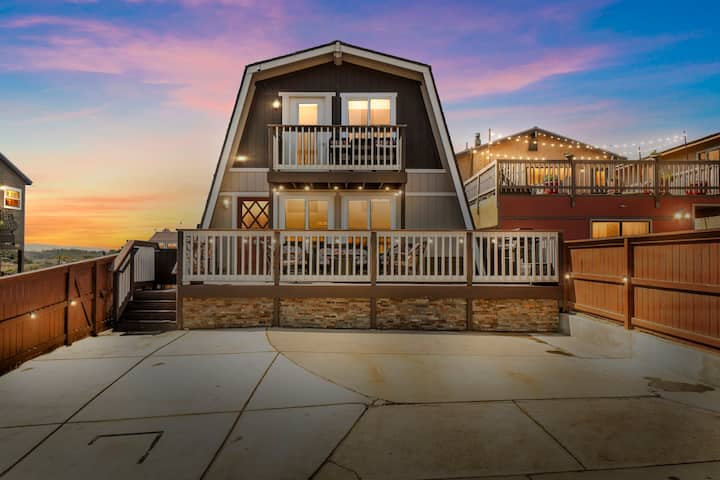This image captures the back of a uniquely shaped two-story house from within a fenced backyard area, characterized by a serene early morning or late evening sky adorned with pink clouds and an orange horizon. The house takes up the center of the wide, vertically-oriented photo, with its dark gray structure contrasted by white wooden trim and rails. The apex of the house features a distinctive, obtuse angle roof that transitions into angled walls, contributing to its unconventional shape.

The foreground reveals a courtyard paved with white and beige stone tiles, leading up to a patio area encased by a white wooden railing. Two large windows and a door are positioned on the ground floor, while steps connect the patio to the courtyard below. The second floor boasts a balcony with the same white railing, accessible through more windows and possibly another door. To the left and right, portions of neighboring houses are visible, completing the residential setting.